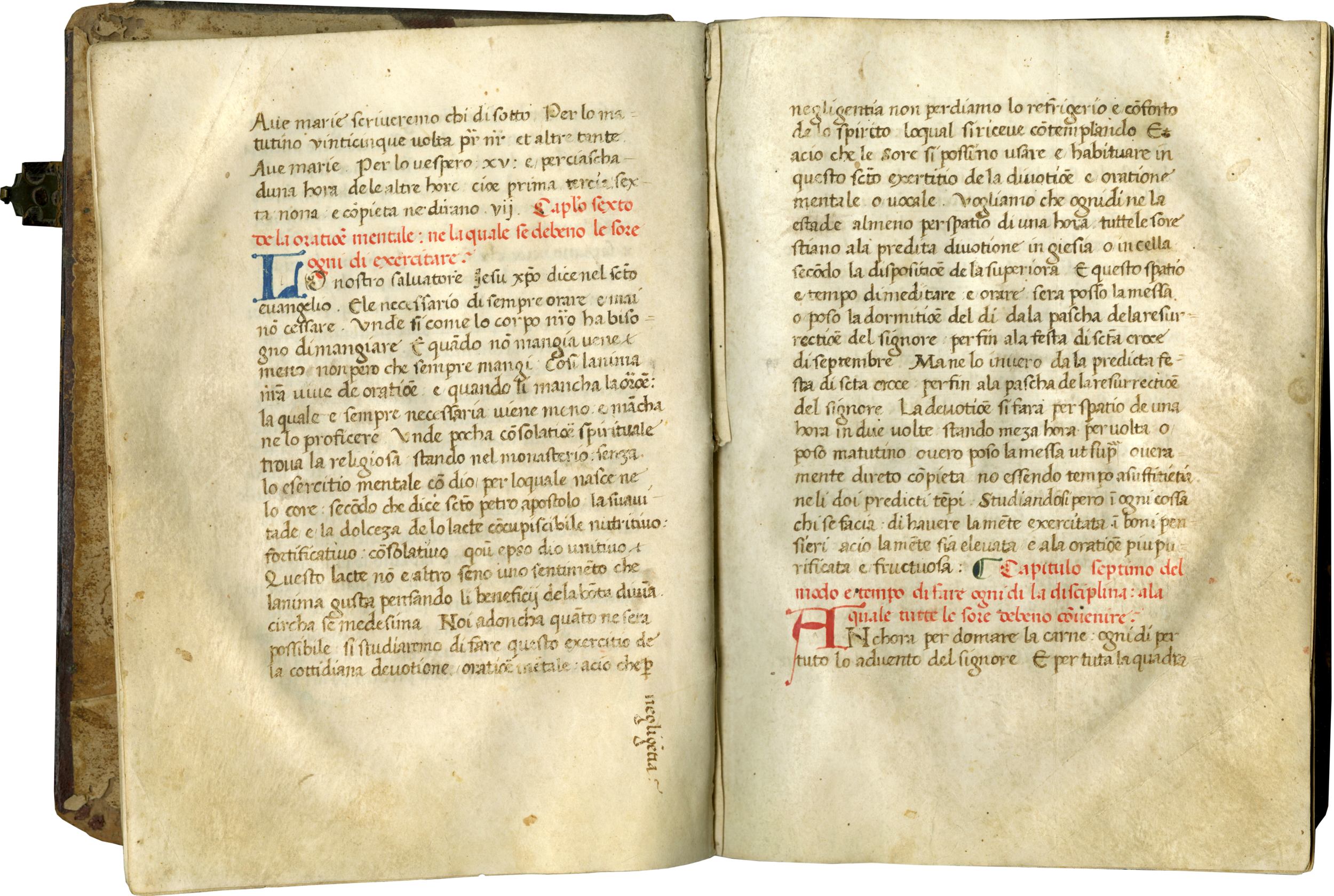The image features a very old, weathered book, opened to reveal its aged, tea-stained pages. Measuring approximately 3 inches high and 6 inches wide when open, the book's leather cover is faded and worn, with visible signs of rot and a metal latch at the top of the left side, suggesting it once had a locking mechanism. The text inside is predominantly in a foreign language, possibly French, written in elegant calligraphy. Both pages contain paragraphs in black ink, punctuated by striking red sentences. The left page features a paragraph beginning with an elaborately colored blue capital "L." Additionally, a noticeable tear in the book's inner seam suggests that a page is missing. The only readable word amidst the ornate script is "Marie," which may refer to a person. The overall impression is of a meticulously handcrafted artifact from a time before modern printing technology.